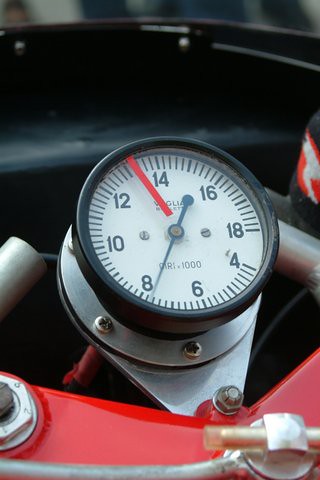A close-up shot of a gauge, likely an odometer or tachometer, enclosed within a vehicle or mechanical setup. The primary color scheme consists of red, black, white, and silver. The gauge displays increments from 4 to 18, marked by even numbers only. It shows a reading of 13, with an additional small dial labeled "Quartz," marked in thousands, and a second hand pointing near 8. The background is blurred with hints of black, indicating the photo might be taken under the hood of a vehicle. The bottom part of the image features a glossy red metallic component secured with a silver bolt with a black top. Emerging from this component is a plastic tube, adding to the overall mechanical context. The picture appears to be taken in daylight.